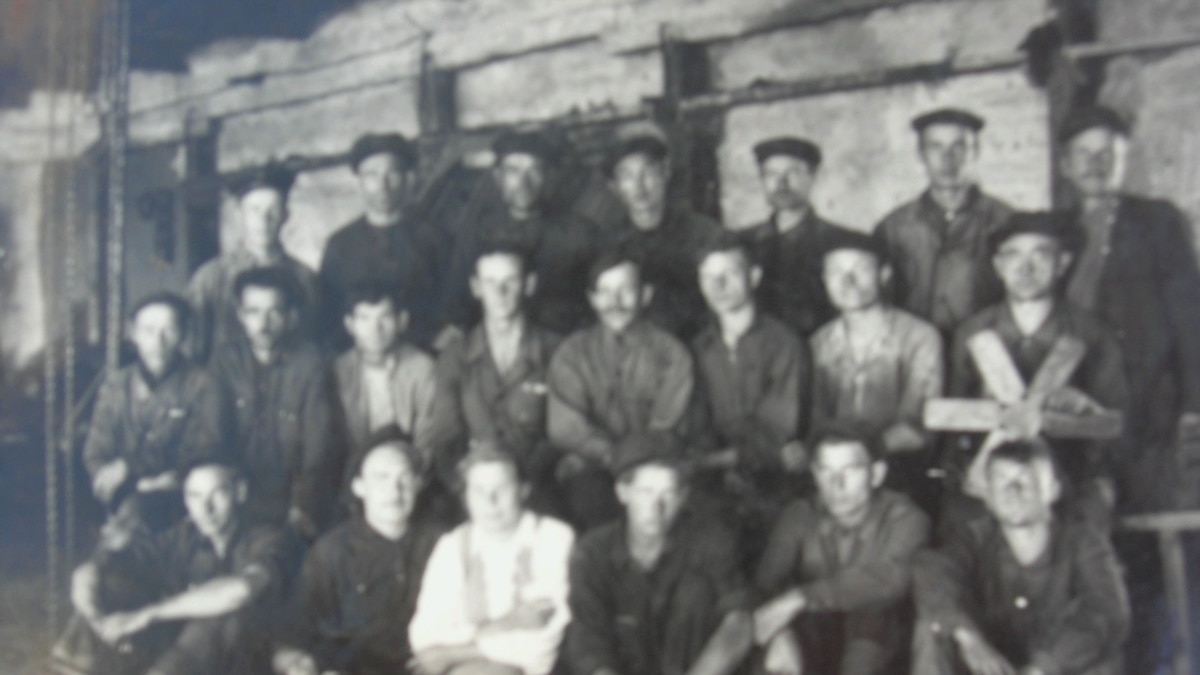This black-and-white, very blurry, historical photograph depicts a group of men posing solemnly and looking directly at the camera. They are either crouched, sitting, or standing in three distinct rows. Most of the men are wearing work uniforms and some kind of old-timey hats or caps, suggesting they are involved in manual labor, possibly coal mining or factory work. One man appears to be holding a propeller-like object. The background hints that they are in a wooden structure, perhaps a warehouse or factory, with visible chains or ropes hanging from the ceiling on the left side and a long rod running behind them on the wall. The photograph carries an air of seriousness, and the men's attire and setting evoke a working-class environment no later than the early 20th century.